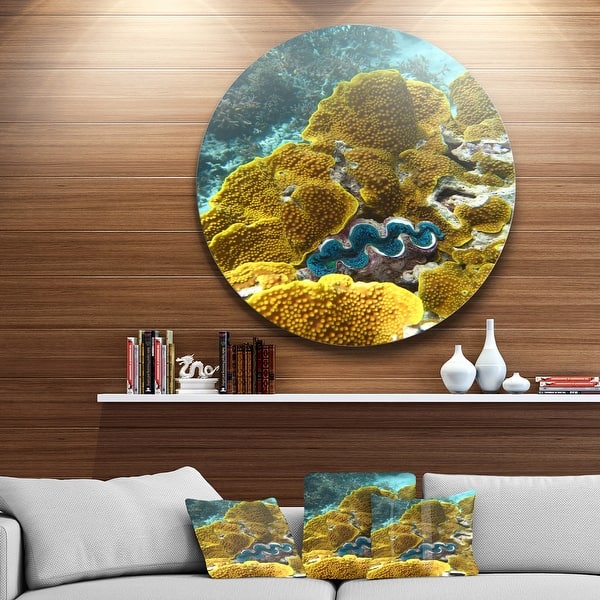The indoor photograph showcases a display room featuring vibrant coral reef designs. Centrally positioned at the bottom of the room is a long gray couch adorned with matching cushions and three throw pillows. These pillows prominently display an identical print of a green coral reef set against light blue underwater surroundings. Above the couch, a wooden wall features a white shelf holding a variety of items: stacked books, a dragon statue, and multiple white vases of varying heights. The shelf supports an oversized round photograph depicting the same coral reef image found on the throw pillows, creating a cohesive underwater theme. Bright lights illuminate the large circular photo, emphasizing its colorful underwater scenery that includes corals and marine plants. The arrangement suggests these elements might have been digitally added to promote the coral reef-themed decor.